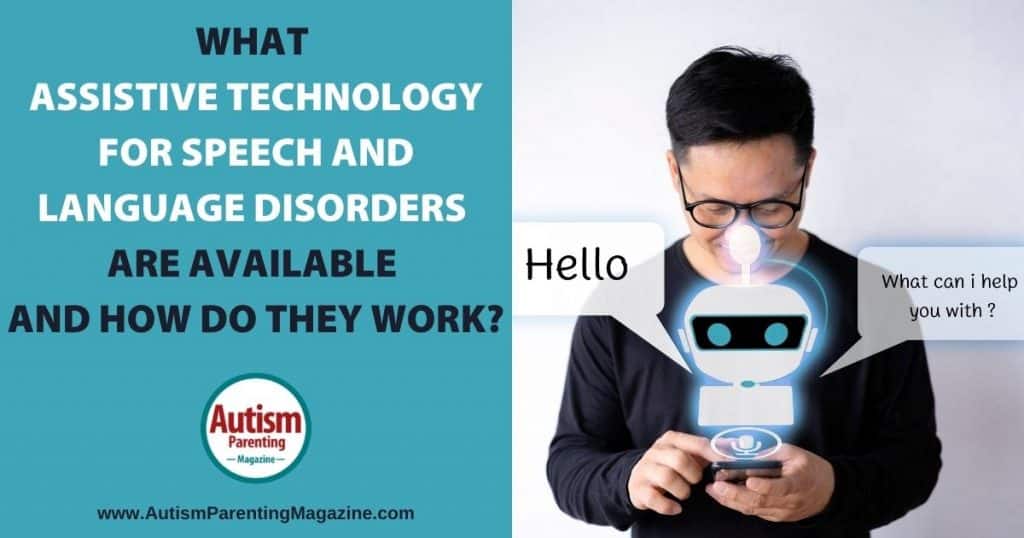This digital poster advertisement from Autism Parenting Magazine is divided into two square sections. The left section has a blue background with centered bold black text that reads, "What assistive technology for speech and language disorders are available and how do they work?" Below this text is a circular logo with a green border and white background. The logo features the words "Autism Parenting Magazine" in red bold letters, and below the logo is the website, "www.autismparentingmagazine.com."

The right section contains an image of a young man with short black hair and black glasses, dressed in a black long-sleeved shirt. He is looking down at a lit mobile device in his hands, from which a robot image is emerging. The robot has a speech bubble saying, "Hello," followed by "How can I help you with?" The background of this section is light gray. This advertisement highlights the available assistive technologies for speech and language disorders, aimed at parents of children with autism.